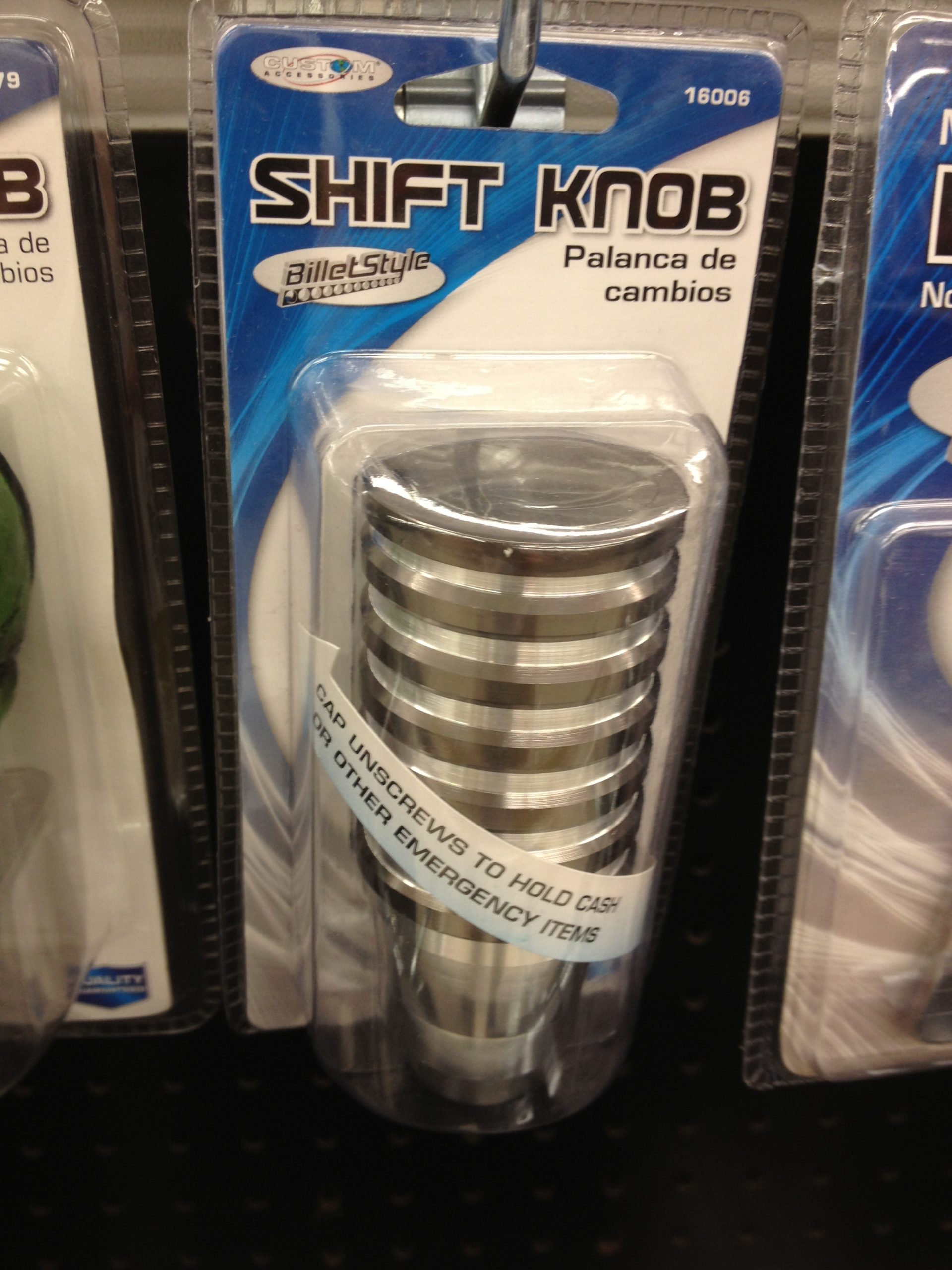The image depicts a packaged shift knob intended for a car gear stick, prominently displayed on a store shelf. Encased in clear plastic packaging with a blue and white design, the shift knob is positioned centrally and slightly towards the top of the image, hanging securely on a hook. The black background contrasts with the packaging's colors: white, blue, gray, red, and silver. The clear container reveals the product’s cylindrical, metallic form beneath. Text on the packaging reads "Shift Knob, Billet Style, 16-006, Palanca de Cambios," with additional information like "cap unscrews to hold cash or other emergency items" displayed across a diagonally placed sticker. The top left corner of the package features the brand "Custom," while the top right corner displays the number "16006." Partially visible neighboring products suggest a well-stocked automotive section in the store.